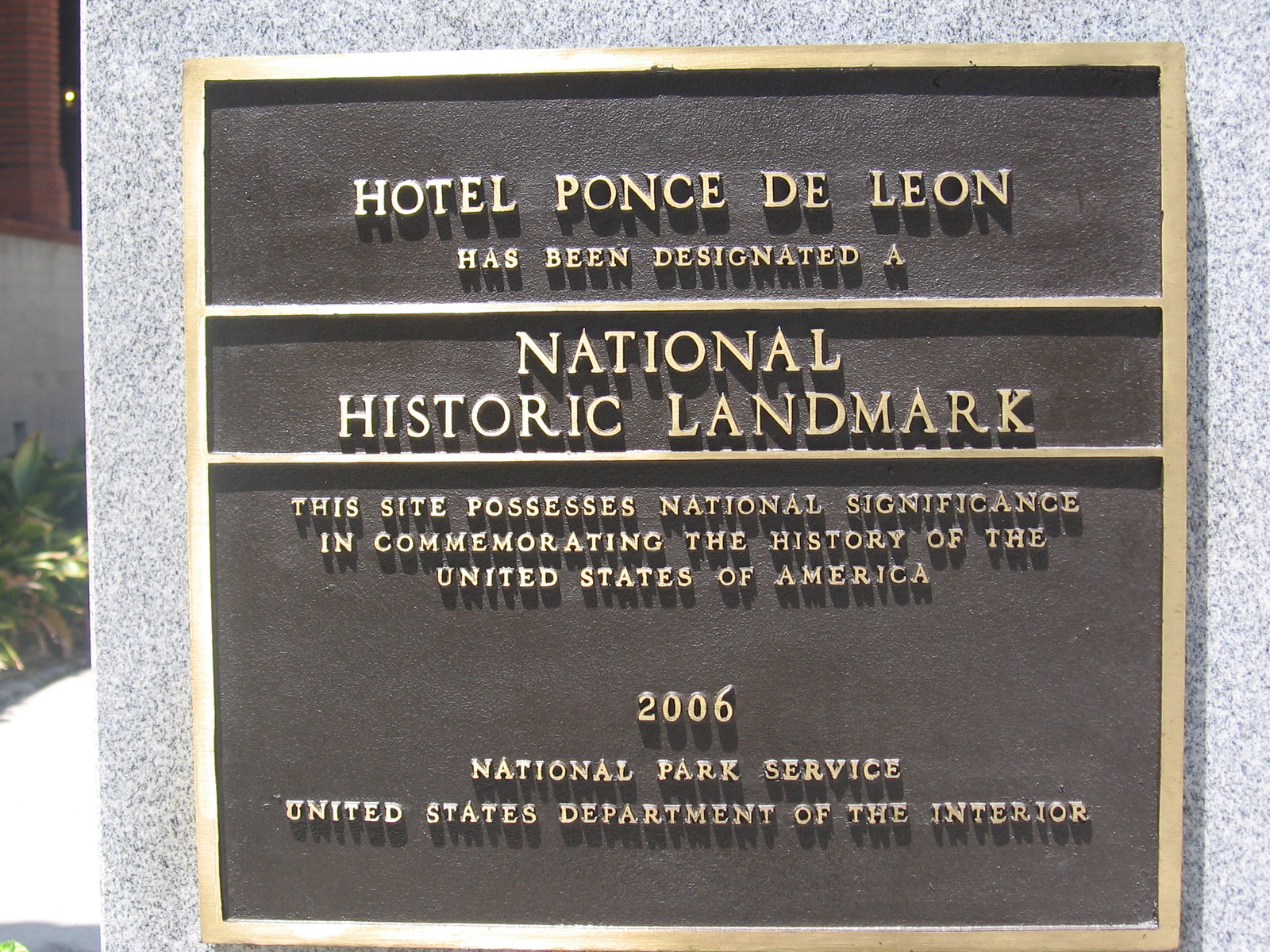The daytime photograph captures a National Historic Landmark plaque mounted on the side of the Hotel Ponce de Leon. The plaque, crafted from bronze, stands out with its polished square shape and shiny letters, contrasting against a rough, textured dark bronze background. The text on the plaque, all in uppercase, reads: 

"HOTEL PONCE DE LEON" at the top, followed by, "has been designated a" below, and then, framed between two horizontal bronze bars, "NATIONAL HISTORIC LANDMARK." Under this central section, the text continues, "This site possesses national significance in commemorating the history of the United States of America." At the bottom, separated by a small gap, it reads, "2006 National Park Service, United States Department of the Interior."

The plaque is mounted on a light gray, speckled granite or marble wall. The sunlight from the left creates a bright reflection along the side of the plaque, emphasizing its polished sheen. The overall style of the image is photographic realism, with the plaque nearly filling the landscape-oriented frame and providing a clear, straight-on view of the historical marker.